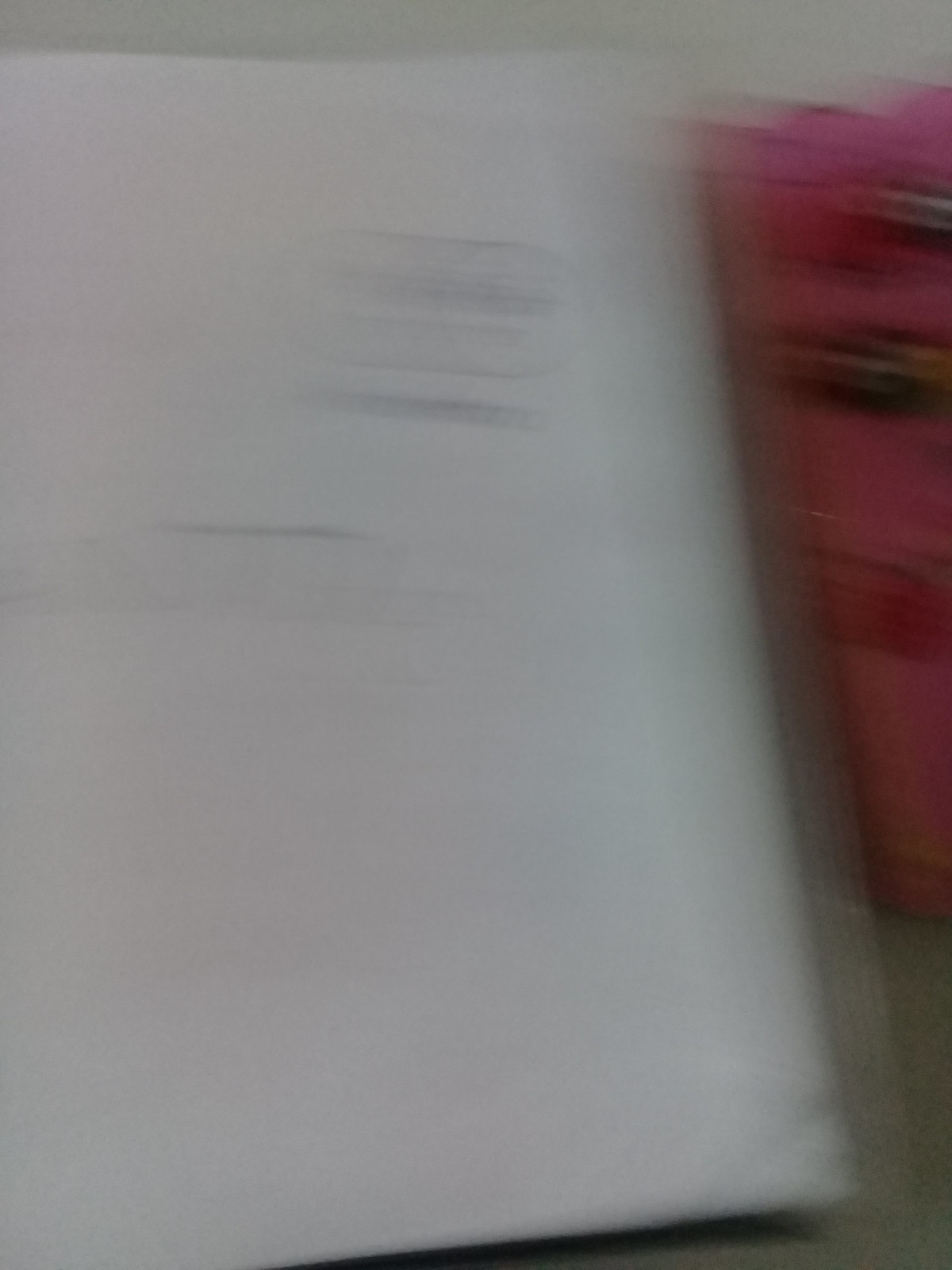This photograph, presented in a portrait orientation, features a primary backdrop of light gray. Dominating the frame is a large, nebulous white rectangular form. The image suffers from significant blurriness, making it challenging to ascertain the nature of this object. However, discernible towards the top right of this white mass are several dark gray lines. Adjacent to the white object on its right side lies another intriguing element; a pink-hued entity marked by a few spots in a blackish-red shade. This pink object is in direct contact with the white rectangular form, adding a layer of mystique to the overall composition.